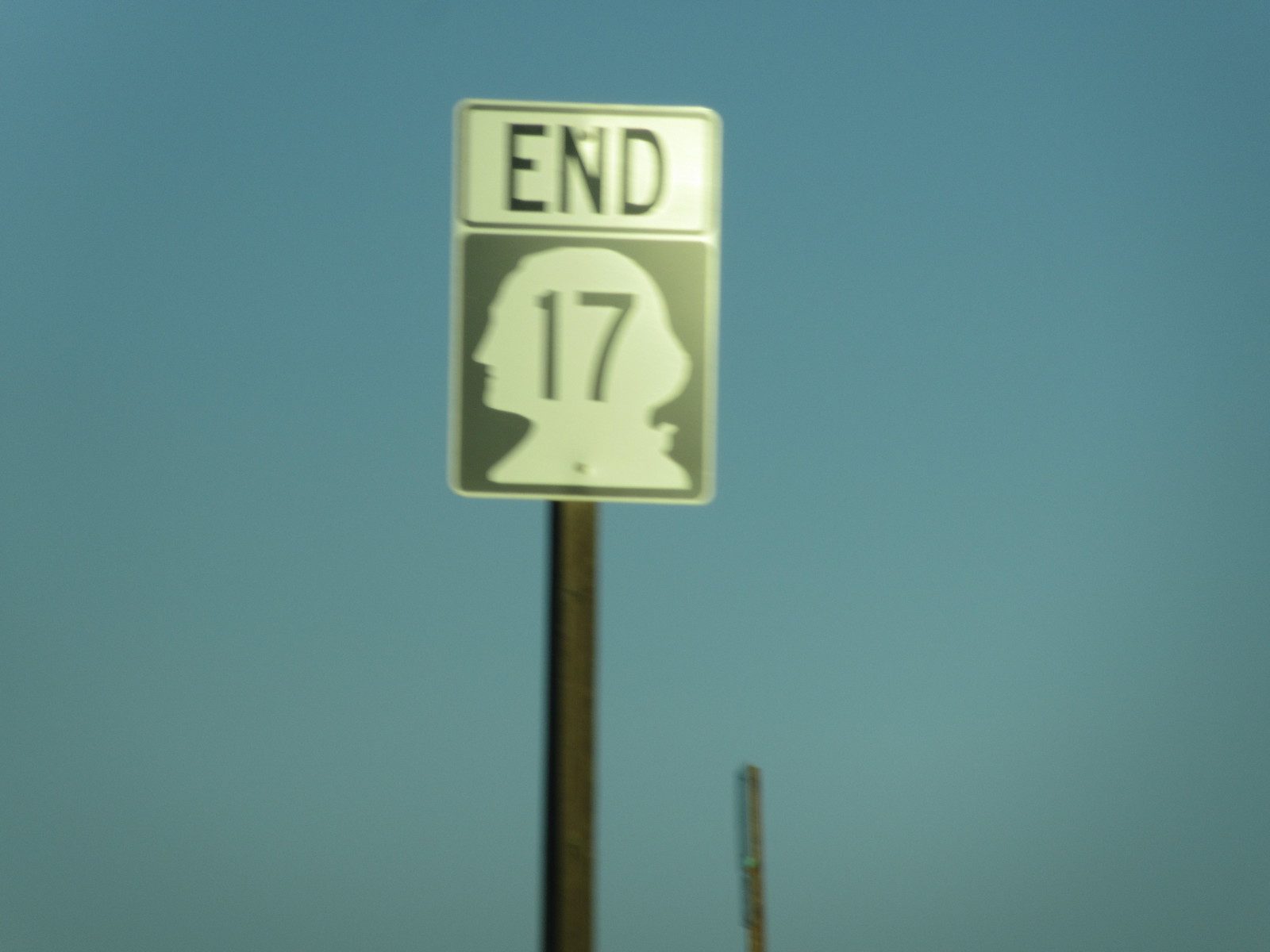This image depicts a street sign, slightly blurry, against a clear blue sky. The sign, mounted on a reddish metal post, is rectangular with slightly rounded edges. At the top of the sign, within a black-outlined area, is the word "END" in black text. Below this, there is a black section featuring a white silhouette of George Washington's head in profile, alongside the number "17" also in black text. Another dark gray post is visible in the background, slightly obscured and lacking any noticeable wires, which adds a sense of depth to the image.